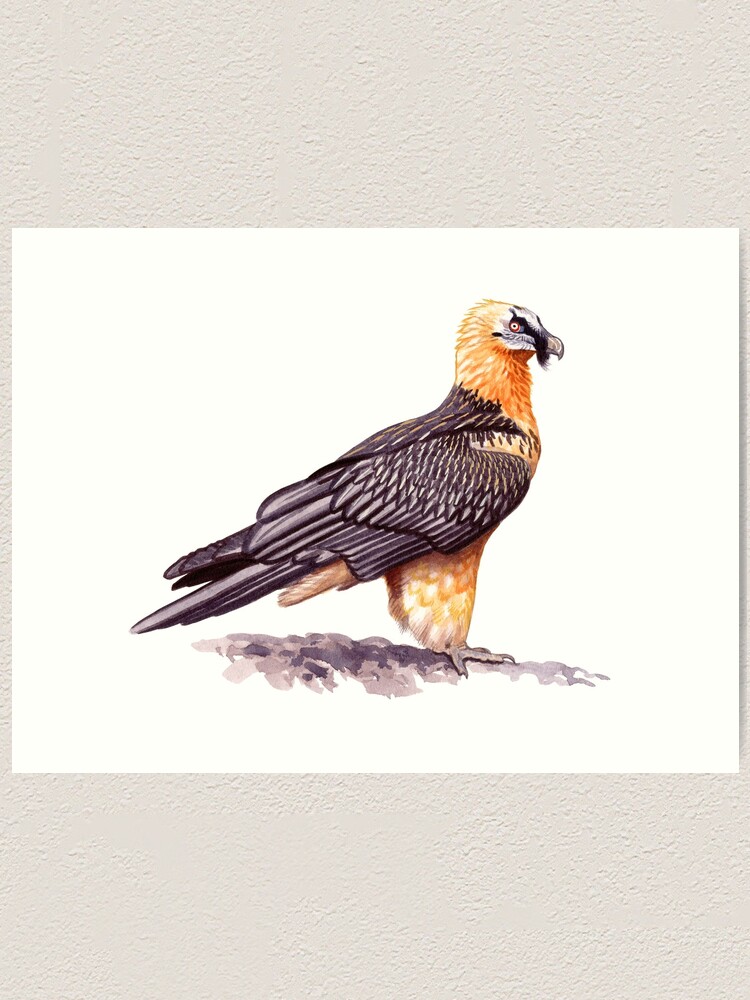This is a richly detailed color watercolor painting of an eagle-like bird that exudes a striking and exotic elegance. The bird is depicted with predominantly brown wings and tail feathers, contrasted by a golden head and feet, giving it a regal appearance. It has a distinctive black wattle or beard that drapes over its beak, adding an unusual yet captivating element to its visage. The bird is positioned either on the ground or on some rocks, and is portrayed looking off into the distance to the right, evoking a sense of contemplative majesty. The painting is set against a plain white piece of paper that is mounted on a cream-taupe textured wall, enhancing the minimalist and focused presentation of the artwork. The entire composition captures the essence of a bird of prey, its large talons and meat-ripping beak highlighting its predatory nature. The overall scene is in a landscape format, emphasizing the broad and expansive feel of the illustration.